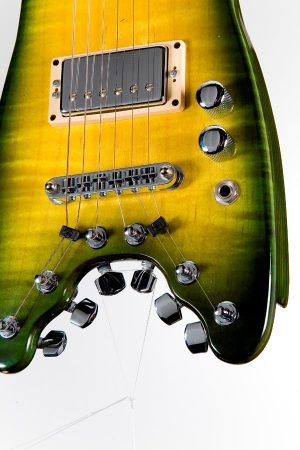The vertically rectangular, full-color photograph showcases a uniquely designed stringed instrument with a six-string configuration, set against an off-white and soft gray-blue background. The instrument, while resembling an electric guitar, displays unconventional features. Its body transitions from a dark green hue on the edges to a vibrant yellow towards the center, with a slightly mottled appearance suggesting a layered paint or stain application. Silver tuning pegs, typically found on the neck, are instead located at the bottom of the instrument. Additionally, the image portrays a silver rectangular component behind the strings, surrounded by white with black screws at the corners. Two silver knobs, capped with black, and a silver input jack for an amplifier are also visible. The detailed craftsmanship of the instrument, along with its distinctive color scheme and inverted string configuration, stands out prominently against the understated background.